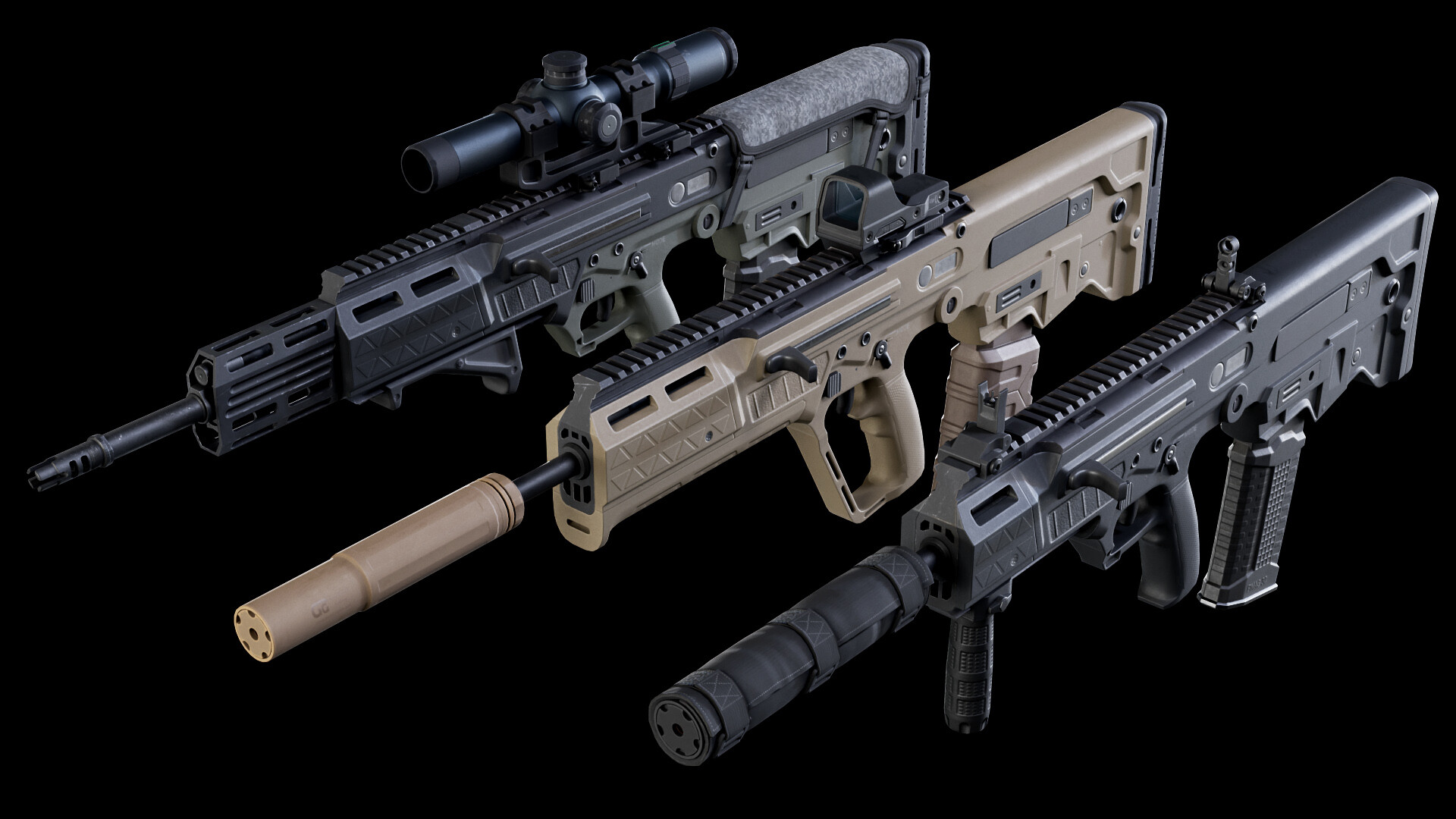The image is a detailed digital rendering of three military-style bullpup rifles arranged diagonally on a completely black background, viewed from above. Each rifle features the compact bullpup design, where the magazine and chamber are situated behind the trigger assembly, making them shorter and easier to handle. The rifles appear to be variations of the same model, distinguished by different configurations and colors.

The rifle on the upper left is primarily black and green, equipped with a long telescopic sight, known as a scope, affixed to the top, and features a brace at the front grip along with a padded stock. The middle rifle is desert tan, outfitted with a boxy red-dot sight and a long cylindrical suppressor over the barrel. The bottom right rifle is all black, with standard metal post sights and a shorter black suppressor on the front. Each rifle has a curved magazine inserted, likely holding 30 rounds, matching the color scheme of the respective rifle. The array of features suggests these representations are sophisticated military issue weapons, presented in different tactical setups.